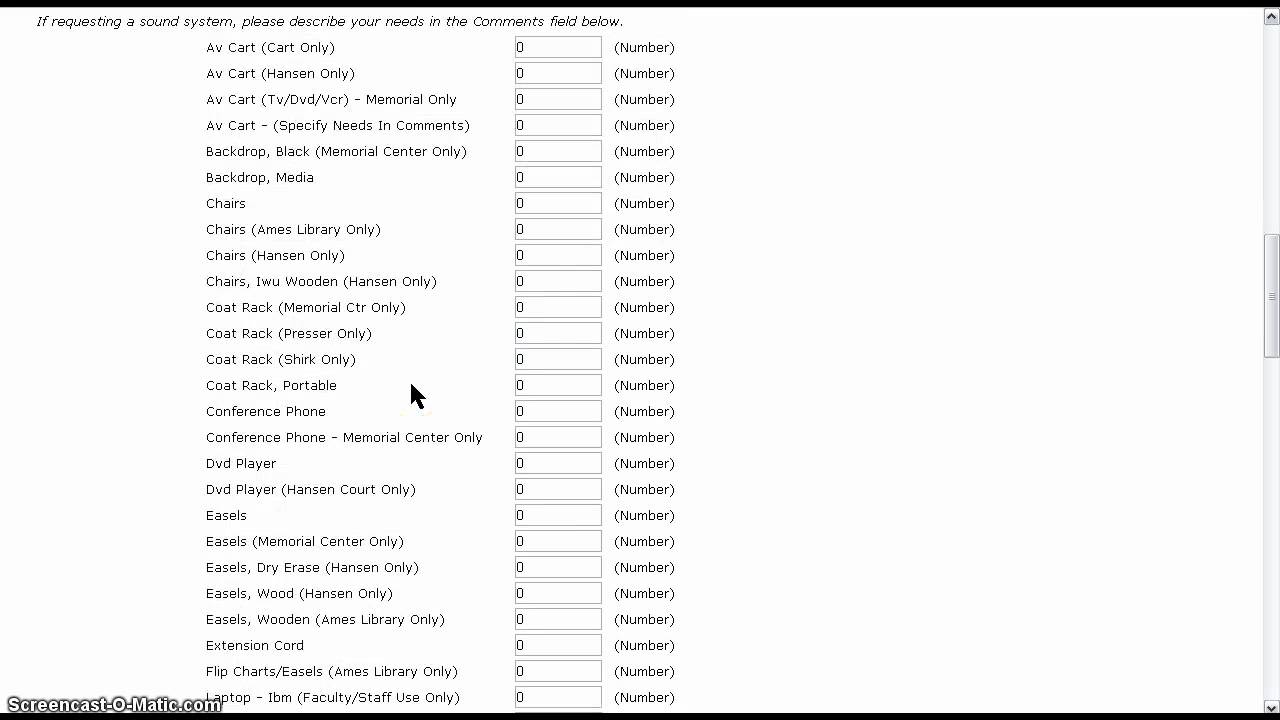The image depicts a white page with a black border along the top, bottom, and left sides. At the top of the page, there is a directive that states, "If requesting a sound system, please describe your needs in the comment fields below." Below this directive is an extensive list of items categorized with various notes and specified locations or conditions for use:
 
1. Comments Field
2. Overlay Information:
   - "L AV cart, cart only: 0"
   - "AV cart, Hanson only: 0"
   - Each entry in the list has an indicator value of 0.
   - Specific mentions include: "AV cart, TV/DVD/VCR Memorial only," "AV cart, specify needs in comments," "backdrop black, Memorial Center only," "backdrop media," and a variety of chair and easel options limited to specific locations such as Ames Library, Hansen, and IWU.
   - Necessary items like a "coat rack, Memorial Center only," "coat rack, Presser only," "coat rack, shirt only," "coat rack, portable," and "conference phone, Memorial Center only."
   - Other equipment including: "DVD player, Hansen court only," "easels, Memorial Center only," "easels, dry erase, Hansen only," "easels, wood, Hansen only," and "easels, wood, Ames Library only."
   - Additional supplies like "extension cord," "flip charts/easels, Ames Library only," and "laptop, IBM for faculty/staff use only."
   
In the bottom left corner of the page, partially overlaying the list, there is a watermark from "screencast-o-matic.com".